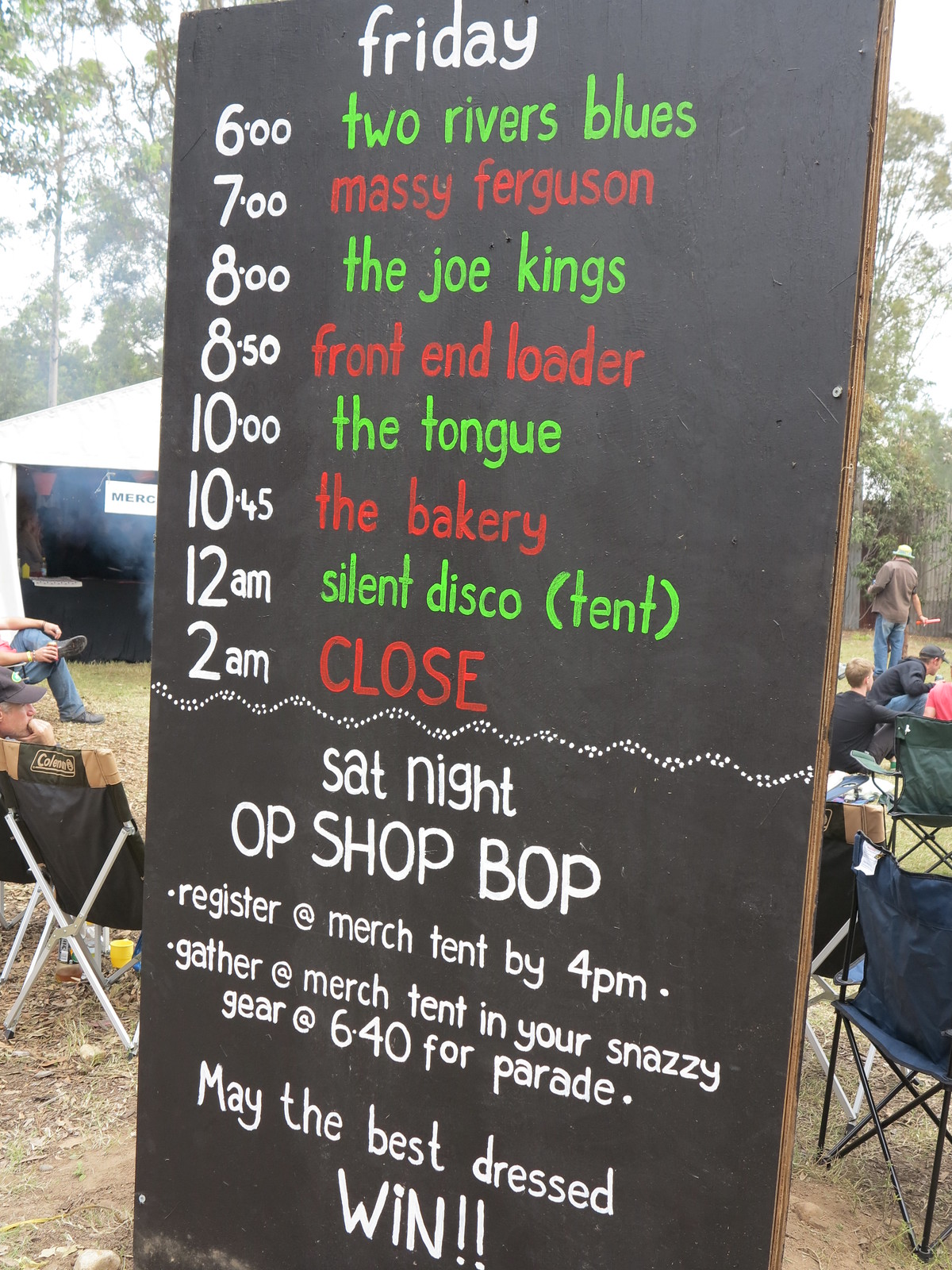The image depicts an outdoor gathering with a central black chalkboard displaying an event schedule. Surrounding the chalkboard are various people seated in camping chairs, including blue and green ones, under a white canopy in the background, indicating a casual festival atmosphere. The chalkboard is old and painted black, with white and alternating green and red chalk details. The text on the board lists events starting with "Friday" at the top, scheduling performances by Two Rivers Blues at 6 p.m., Massey Ferguson at 7 p.m., The Joe Kings at 8 p.m., Front End Loader at 8:50 p.m., The Tongue at 10 p.m., The Bakery at 10:45 p.m., and a Silent Disco at midnight, concluding with a closing time at 2 a.m. Below a curved dotted line, it details "Saturday Night OP Shop-Bop," instructing attendees to register at the Merch Tent by 4 p.m., gather there in snazzy gear by 6:40 p.m. for a parade, with a best-dressed contest. The scene is set on a grassy area with trees in the distance and a mostly sunny sky above, contributing to the lively and communal ambiance.